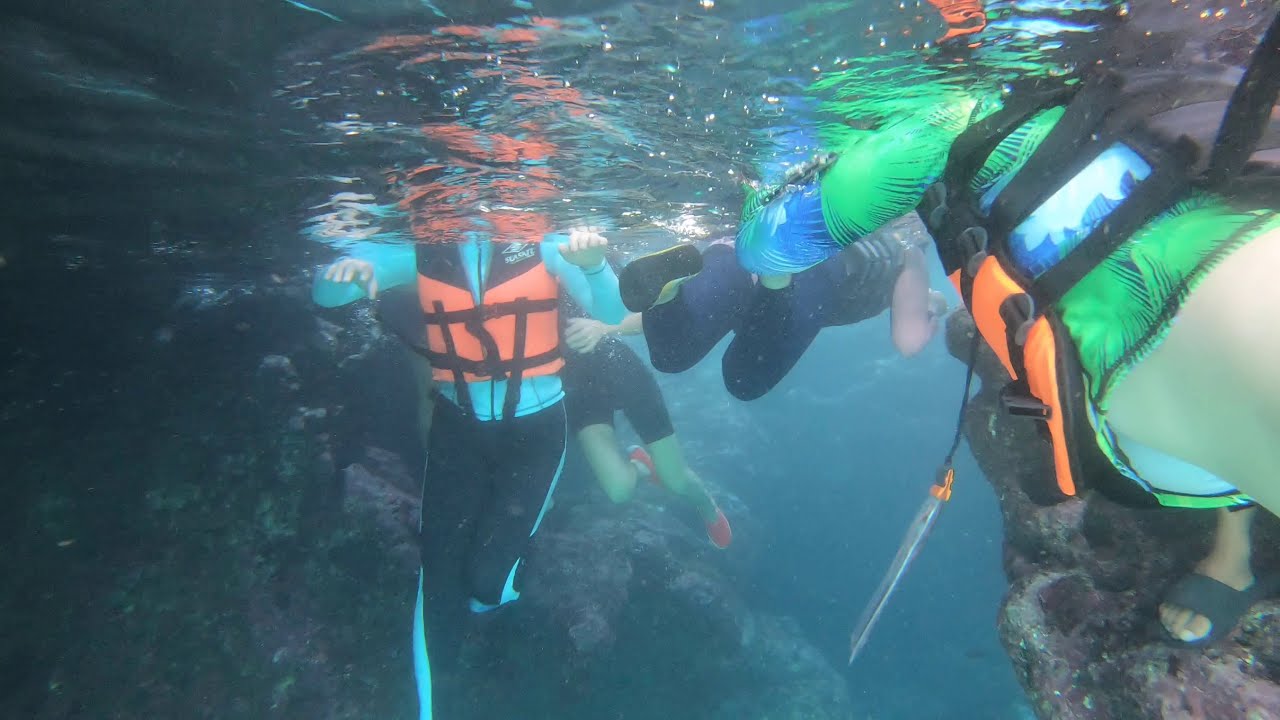The image captures an underwater scene featuring several snorkelers or scuba divers exploring a rocky coral-reef-like environment. The surface of the water is visible at the top of the frame, with light penetrating through, creating a sparkling effect. Approximately five people are visible from the neck down, floating near the water’s surface, their heads breaking through to the air above. They are wearing wetsuits in shades of blue and green, along with bright orange buoyancy vests or life preservers, and flippers. The water beneath the surface appears blue and somewhat hazy, creating a cloudy effect. Around them are large, rocky formations that resemble coral reefs or underwater caves. While most of the visible skin suggests they are white, a brown foot in a sandal hints at some diversity among the group.